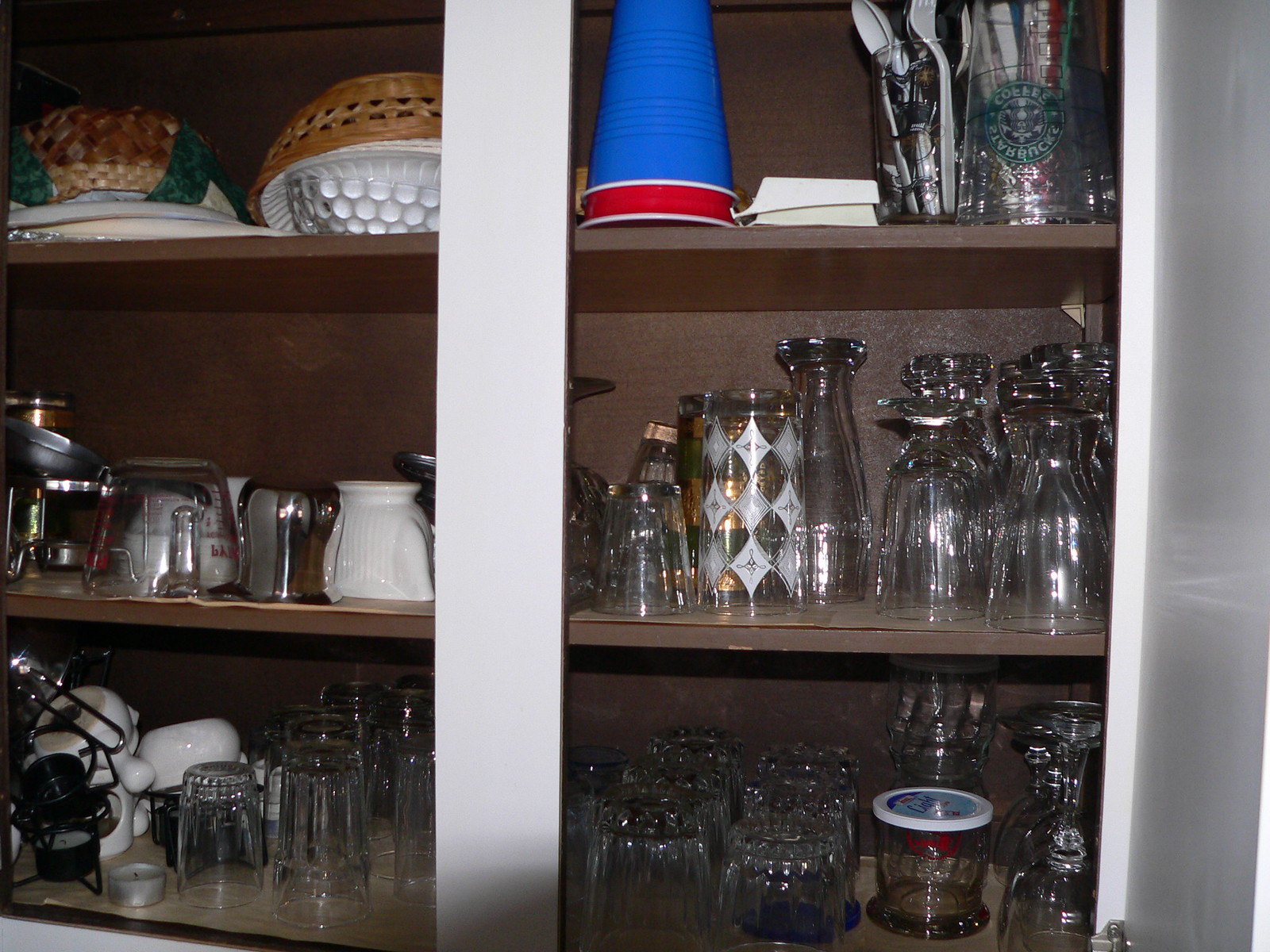A close-up of an open wooden cabinet reveals a blend of rustic and modern elements. The interior surfaces display the natural brown hue of unpainted wood, contrasting with the white-painted cabinet doors. The cabinet is organized into three shelves, each replete with a variety of kitchenware. 

The bottom shelf houses an assortment of crystal-cut drinking glasses and several white plastic kitchen tools. On the middle shelf, to the left, a glass measuring cup is stationed beside an array of drinking glasses and beer tumblers, arranged meticulously. The top shelf showcases an eclectic mix of decorative bowls in white and brown, alongside a red and a blue disposable cup. Additionally, this shelf contains a set of plastic forks and spoons, rounding out the diverse collection.